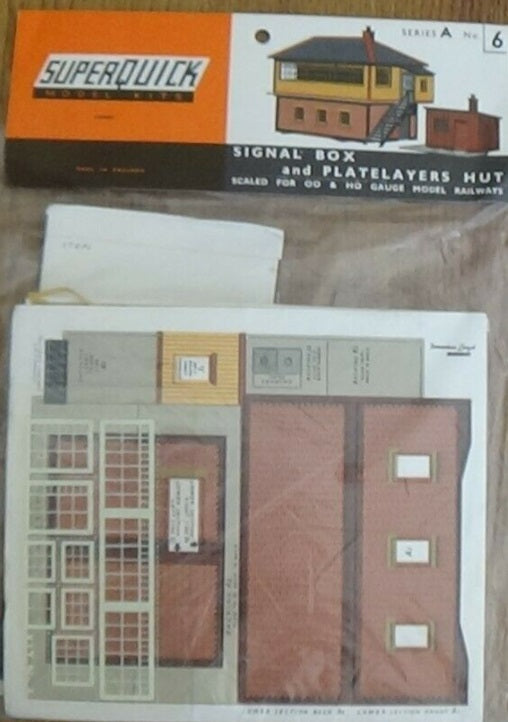This image features a packaged model kit for a miniature scene, likely intended for model train enthusiasts or architectural hobbyists. Encased in a clear plastic product bag with a cardboard header, the kit includes cardboard cutouts to assemble a three-dimensional signal box and a platelayer's hut, both typical of railway settings. The cardboard header, designed for hanging on a store shelf peg, bears the "Superquick" brand name against an orange background. The kit appears to be an older product, indicated by the blurry, low-quality image resembling a photo taken with an older camera. The content inside the package is flattened for display and shows an illustrated depiction of the assembled pieces, highlighting the final two-story signal box structure. No additional text is visible in the image.